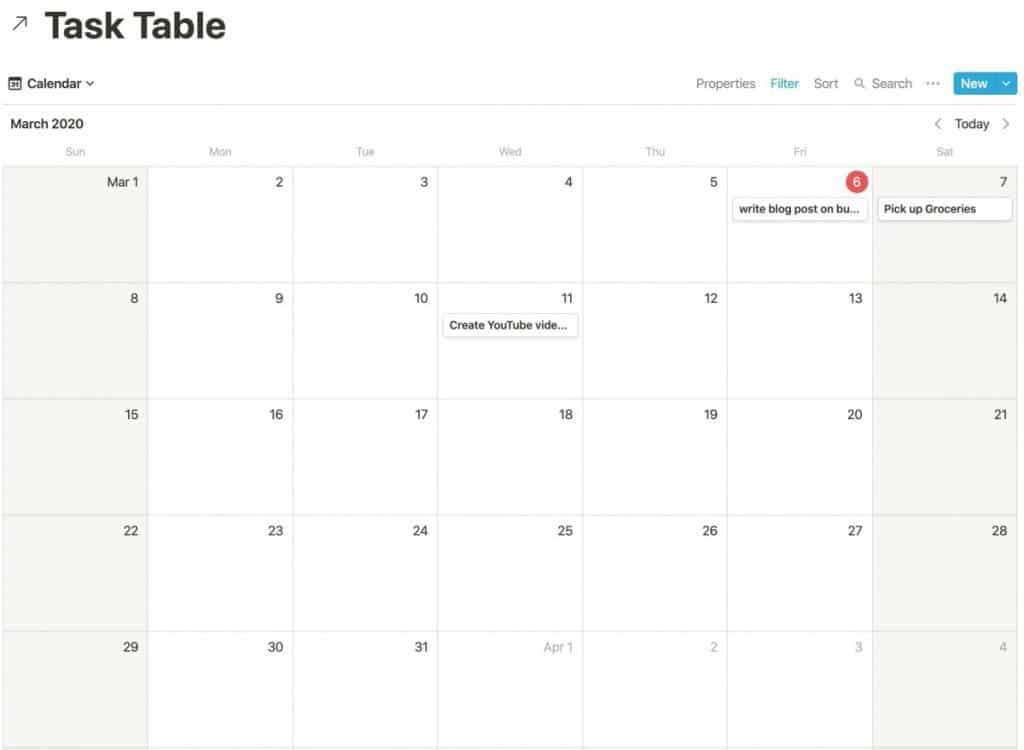In this image, a calendar for the month of March 2020 is prominently displayed against a primarily white background. The upper left corner features a task table labeled "Task Table." Meanwhile, the upper right corner contains options for "New," "Properties," "Filter," "Sort," and "Search." Specific dates have been populated with tasks: "Rise Blog Post" is scheduled for March 6th, "Pick Up Groceries" for March 7th, and "Create YouTube Videos" for March 11th. The remaining days of the month are devoid of any entries.